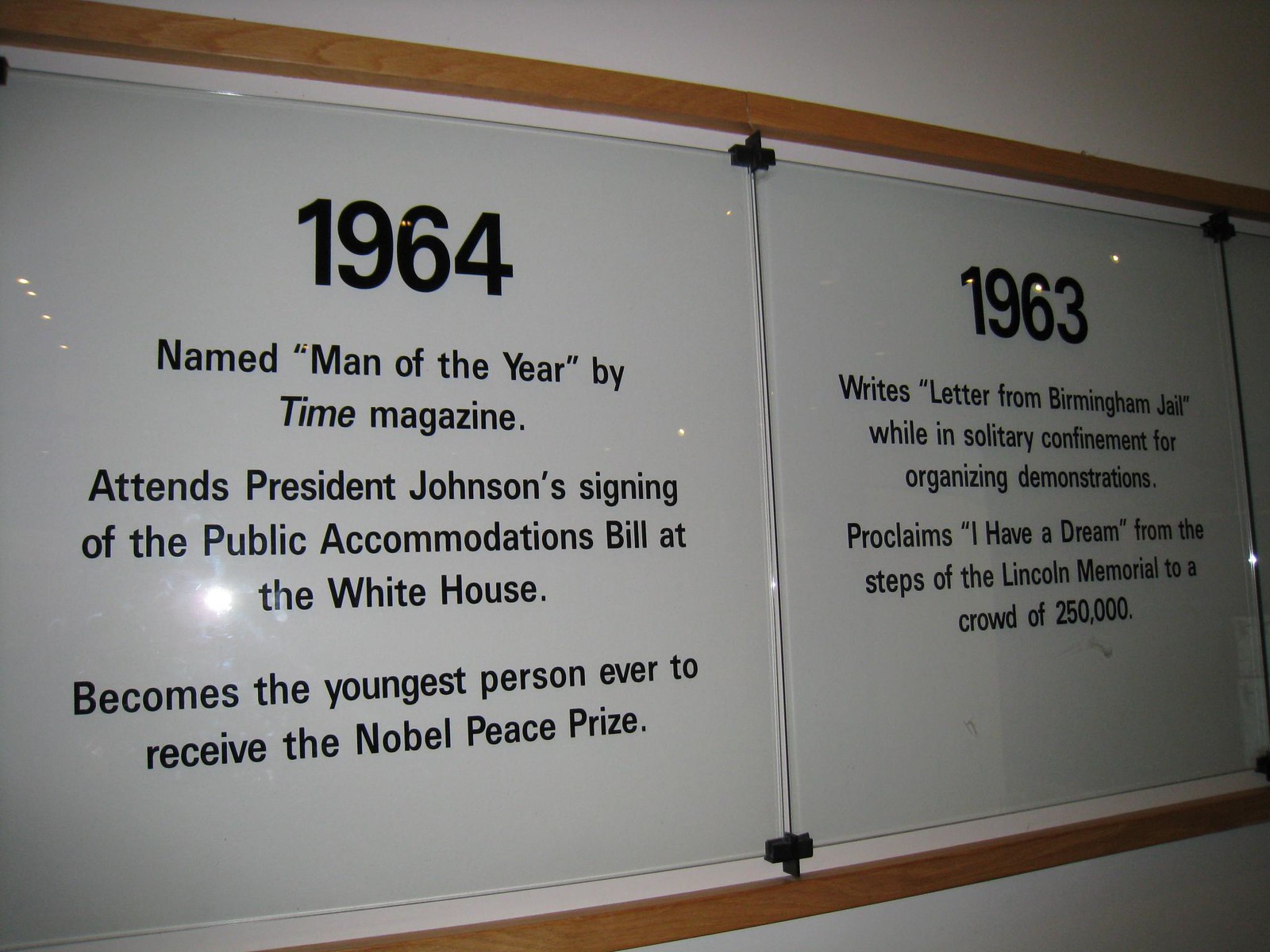The image depicts a horizontal signboard mounted on a white wall, framed with a wooden border and featuring two glass panels side by side, reflecting light from the opposite side. The signboard documents a historical timeline of Martin Luther King Jr.'s achievements, presented in a photographic and representational style.

On the left glass panel, bold black letters at the top read "1964." Below this, in black text, it states: "Named 'Man of the Year' by Time magazine. Attends President Johnson's signing of the Public Accommodations Bill at the White House. Becomes the youngest person ever to receive the Nobel Peace Prize."

The right glass panel is similarly formatted, featuring "1963" in bold black letters at the top. The text underneath reads: "Writes 'Letter from Birmingham Jail' while in solitary confinement for organizing demonstrations. Proclaims 'I Have a Dream' from the steps of the Lincoln Memorial to a crowd of 250,000."

The plaques are encased in glass fitted into the wooden frames with black attachments, showcasing significant milestones in Martin Luther King Jr.'s life.